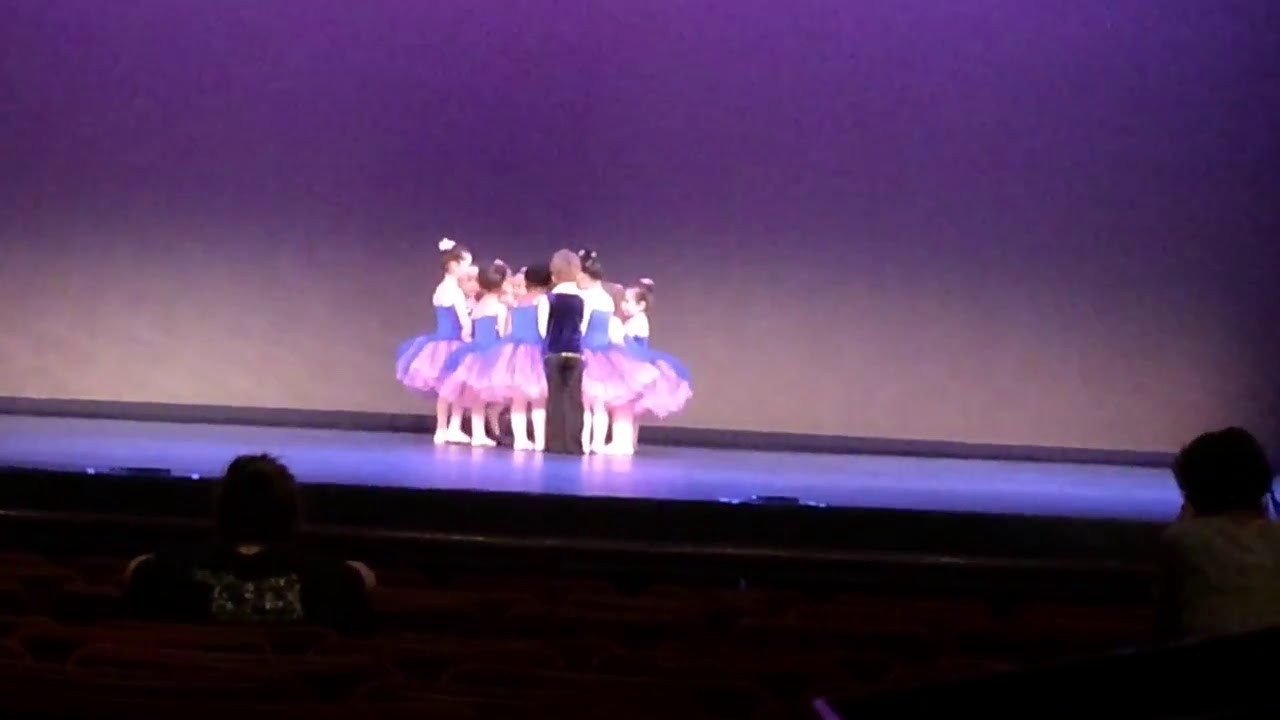The photograph captures the view from within a dimly lit theater or auditorium, showcasing an audience's perspective. At the forefront, the backs of two audience members' heads are visible in the darkness, highlighting the deep, obscured rows of reddish auditorium chairs. The stage commands attention with its vibrant lighting, revealing a distinct blue floor and a backdrop that transitions from a darker purple to a soft lavender hue near the bottom.

Center stage, a group of children stand in a circle, seemingly poised to perform. The young girls are dressed in charming ballerina outfits, characterized by purple or bluish-purple tops and fluffy pink tutus, complemented by white stockings. Their hair is neatly styled in tight buns, adorned with ornaments. Among them, a boy with reddish hair stands out, wearing a purple velvet vest over a white shirt, paired with black pants. The children, with their backs to the audience, form a picturesque circle, ready to enchant with their performance.